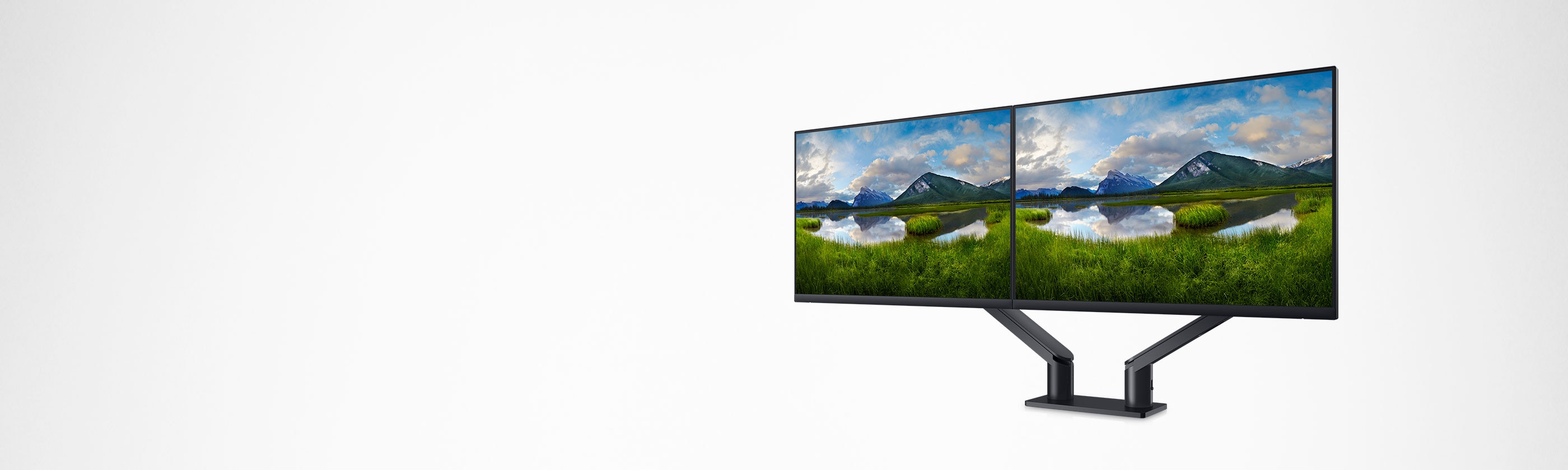The photograph depicts a dual monitor setup mounted on a single stand, which is centrally positioned against a white backdrop with subtle shading on the left side. The stand itself features two diagonal arms extending to hold each of the fairly large monitors. The base of the stand is a rectangular shape, connecting to a cylindrical support. Both monitors are angled slightly diagonally inward and display identical wallpaper images. The wallpaper illustrates a lush grassy area in front of a tranquil body of water, with a majestic mountain range in the distance, topped with hints of snow and under a sky filled with clouds. The scene is serene and natural, lending a cohesive aesthetic to the dual screens within the minimalist composition.